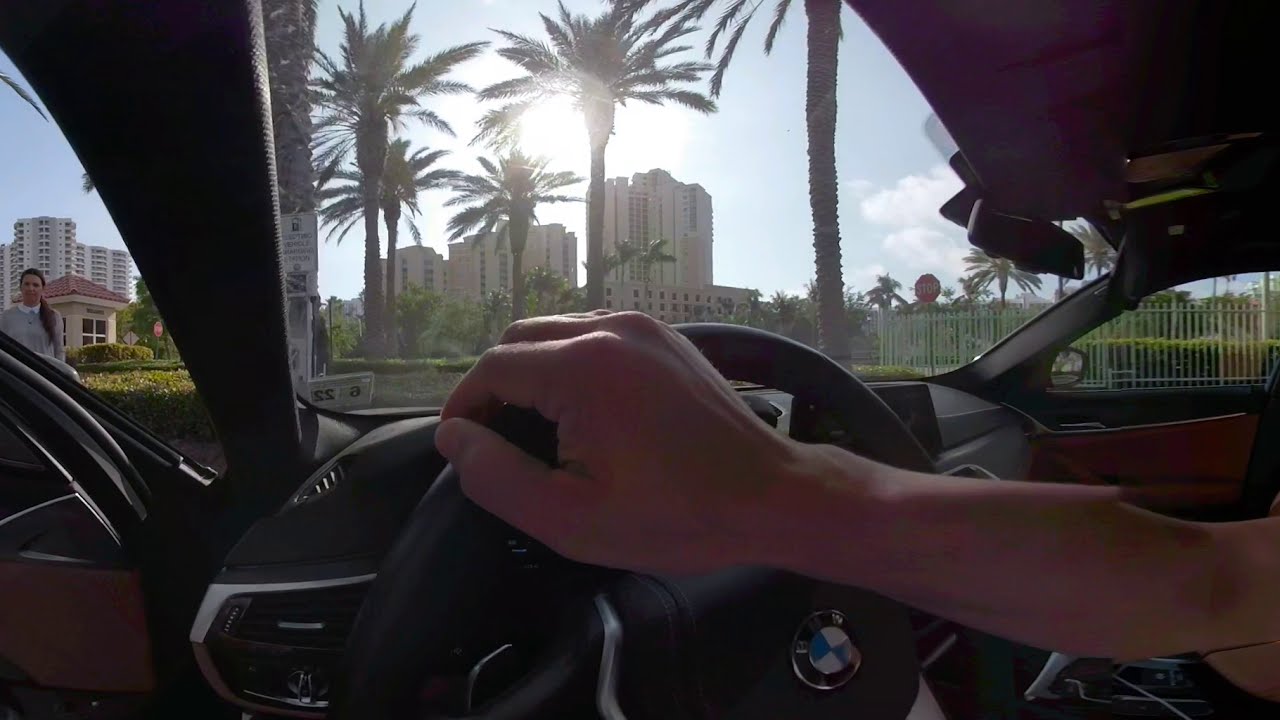The image depicts a man inside a BMW with a black interior and brown trim, taken from the left of the driver. His right hand rests at the top of the steering wheel, and the driver's door is open, suggesting he is about to meet the girl visible in the left corner of the frame. The girl, wearing a blue dress and a white collar with her ponytail draped over her right shoulder, stands beside the car looking at the driver. Sunlight streams through the windshield, illuminating the scene and highlighting six tall palm trees and a red stop sign, indicating a likely tropical U.S. location. The background features tall square buildings, about 15 to 20 stories high, including one with a round tower, all under a bright, clear blue sky. The image captures a moment rich with detail, from the car's luxurious interior to the vibrant urban and tropical environment outside.